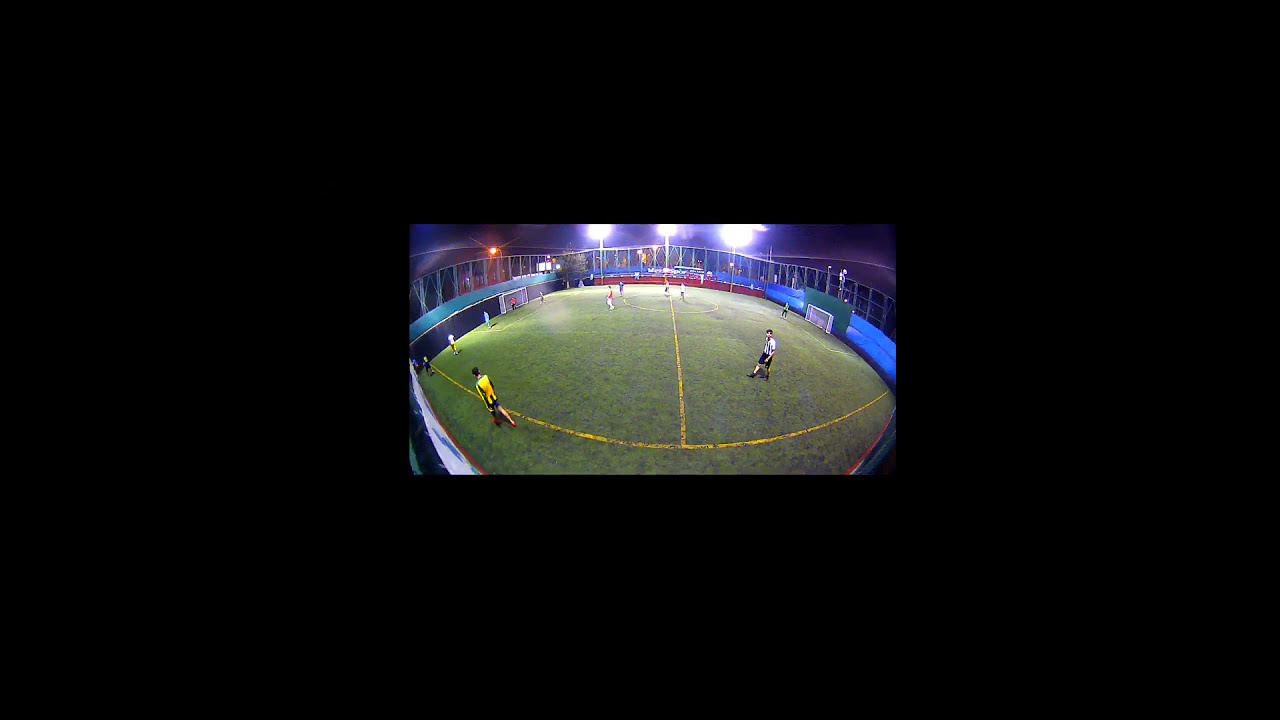The photograph showcases a nighttime outdoor soccer game on a small, fenced-in pitch with artificial green turf, marked with distinctive yellow painted lines. The image, framed by a thick black border on all sides, gives a fishbowl effect, adding a rounded perspective to the rectangular outline. Despite the dark night sky in the background, the field is brightly illuminated by three prominent stadium lights positioned at the top of the image. The scene captures around ten players, with the right side showing a player in a white shirt and black shorts, and the left side a player in a yellow shirt. The pitch is set up for a small game, possibly three-on-three, with goals on both ends. The seating area surrounds the field, with the stadium walls featuring blue and red hues. The midfield line and a large circle encompassing it are also evident, though no soccer ball is currently visible on the field.